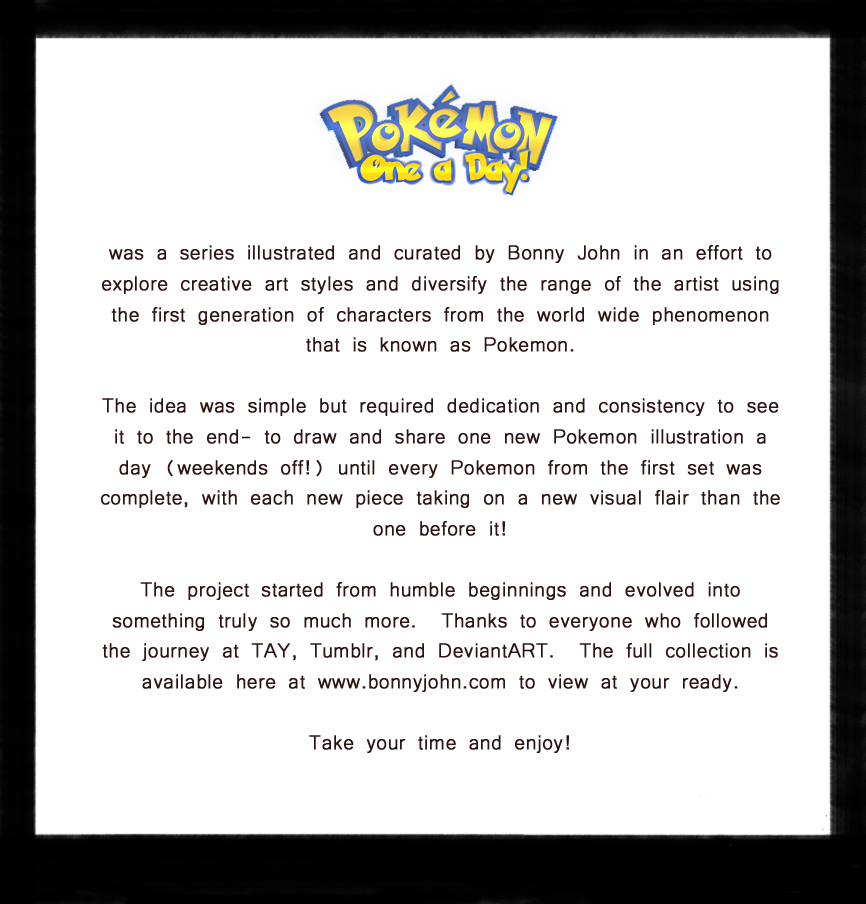An image with a thick black border encasing the entire frame presents a striking and minimalist design. The background is pure white, with no additional images or illustrations. Near the top center, prominently displayed, is the iconic Pokémon logo. Directly beneath it, the phrase "One a Day!" is featured in bold text. Following this, the main content is divided into a few neatly organized paragraphs.

The first paragraph introduces the series, which was illustrated and curated by Bonnie John. It explains that the project was an effort to explore creative art styles and diversify the artist’s range by using characters from the first generation of the globally renowned phenomenon, Pokémon.

The second paragraph elaborates on the project's premise. It describes the simple yet demanding goal of creating and sharing one new Pokémon illustration each day, with breaks taken on weekends. Each new illustration embodies a distinct visual flair, ensuring a fresh and diverse approach to every character until the entire first set of Pokémon was completed.

The third paragraph reflects on the project's growth from its modest beginnings. It acknowledges the support and engagement from followers on various platforms such as Tay, Tumblr, and DeviantArt, and invites viewers to explore the full collection available at www.bonniejohn.com. The paragraph conveys gratitude and an appreciation for the community that followed the journey.

Concluding the text, a final centered sentence invites viewers to take their time and enjoy the collection.